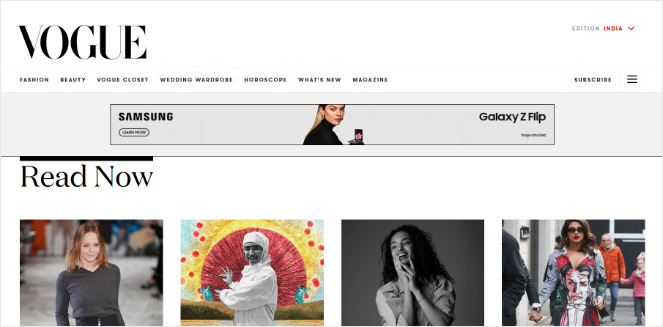The screenshot captures the Vogue magazine website. Prominently positioned at the top left is the iconic Vogue logo. Directly beneath it, an organized row of tabs spans across the page, labeled sequentially as Fashion, Beauty, Vogue Closet, Wedding Wardrobe, Horoscope, What's New, and Magazine. To the right of these tabs, there is a section encouraging visitors to subscribe, marked by three small words and four vertical lines.

Below the navigation tabs is a large advertisement for the Samsung Galaxy Z Flip. The ad features a sophisticated image of a woman in a black turtleneck gracefully holding up the phone. Following this advertisement is a section titled "Read Now," presenting four distinct images that likely correspond to four different articles available on the site. The layout is clean and visually engaging, guiding the reader effortlessly through various content sections.